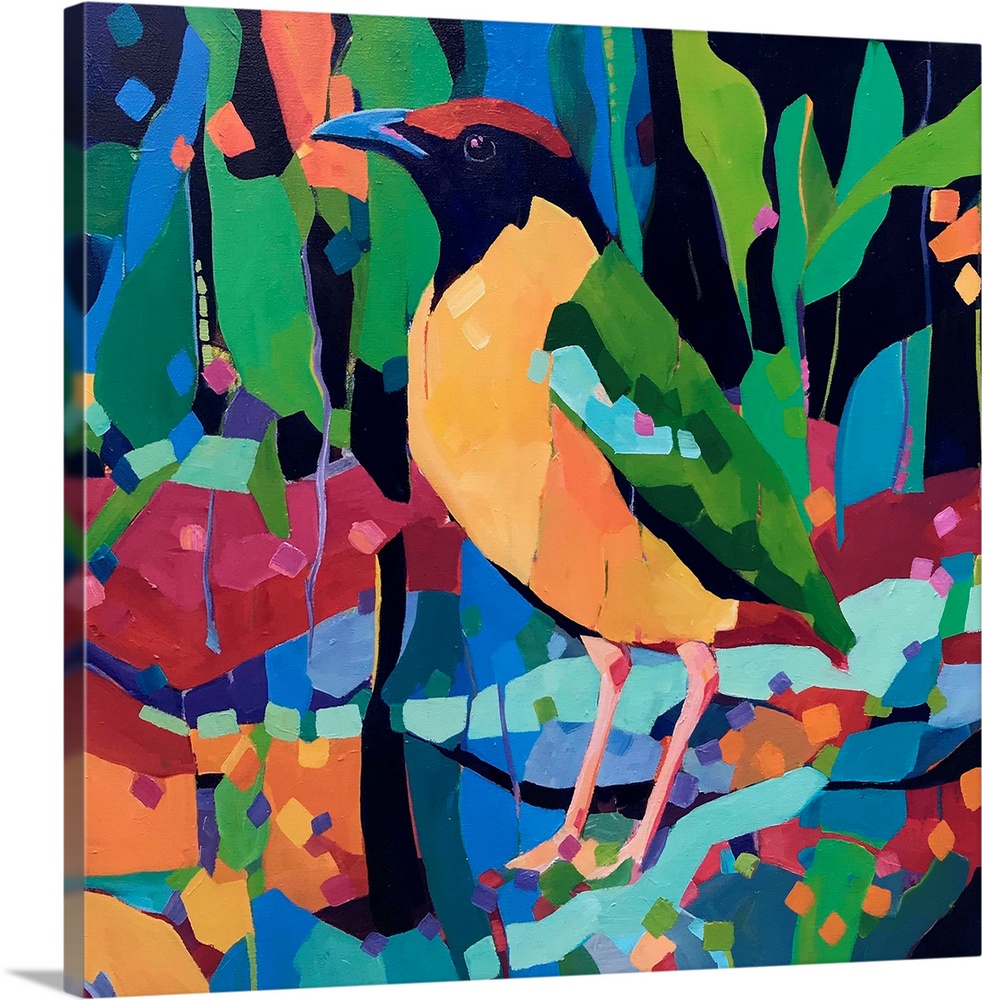This artwork, an oil painting on canvas, depicts a vibrant bird centrally positioned. The artist extended the colors and patterns onto the edges of the canvas, creating a seamless, immersive effect. The bird is striking with a yellow breast, a black lower head, and a red crown. Its beak is predominantly blue with hints of pink, and its eye features a blend of pink and white. The bird's wings are predominantly green, accented with blue and black, while its tail feathers are red. The legs of the bird show a mix of pink and red hues. Behind the bird, a backdrop of leaves and a patchwork of multicolored squares evoke a jungle atmosphere. The painting is characterized by flat, bold colors without gradient shading, enhancing its vibrant, mosaic-like appearance.